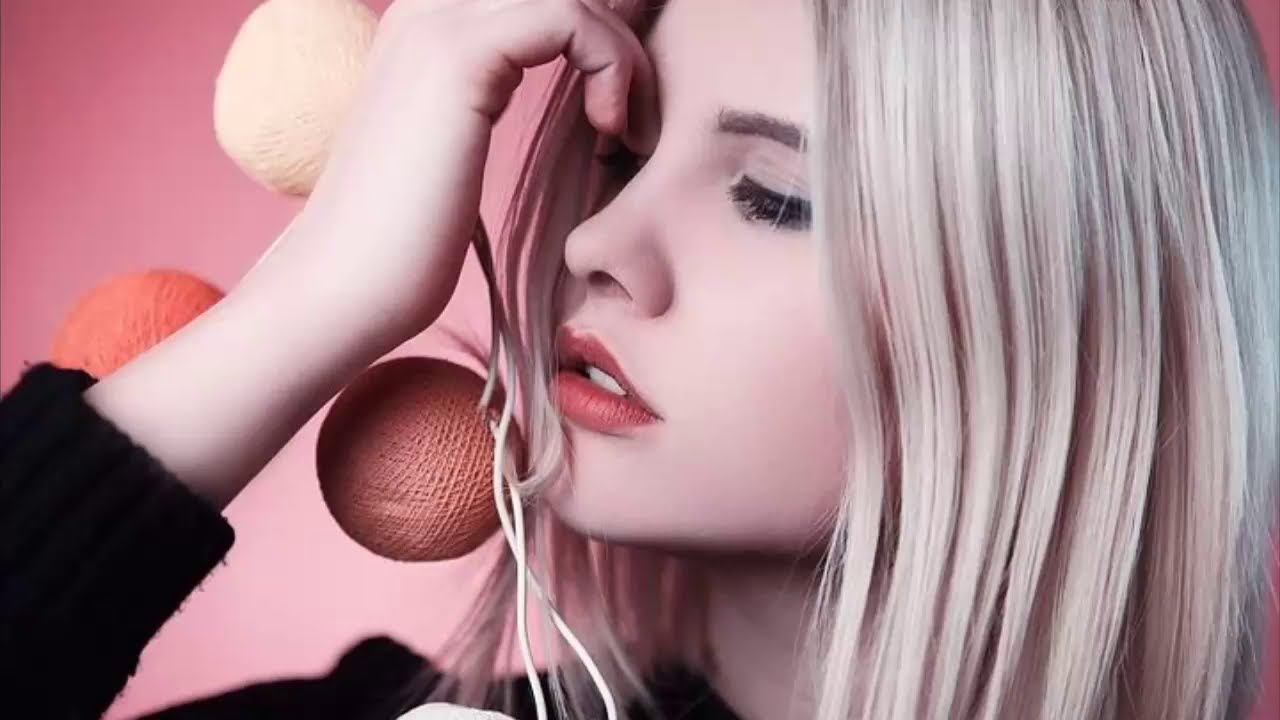In this detailed image, we see a blonde-haired female model with dark, trimmed eyebrows and long eyelashes, wearing red lipstick. Her hair, parted to the side, cascades down and partially covers her face as she looks off to the left, eyes closed. Her fair complexion is accentuated by a black sweater. The model's right hand is raised, seemingly moving her hair away from her face or possibly holding three perfectly wound balls of string. These balls – in shades of light white, orange, and a reddish-tan – appear suspended in midair towards the top left of the image. Two white strings connected to these balls hang down, possibly held by the model but their exact origin remains unclear. The entire scene is set against a pink background, and the overall composition suggests a stylized photoshoot, likely intended for a social media post or a modeling portfolio.